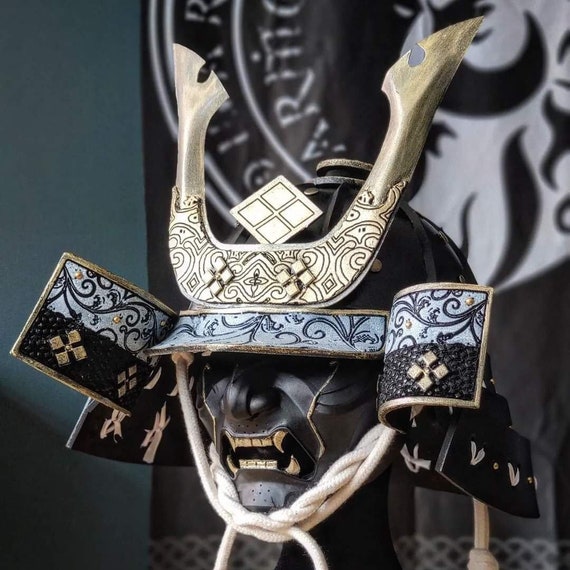The photograph showcases a detailed, samurai-inspired warrior mask that appears ancient, with a fusion of various cultural artistic designs. The predominantly black helmet features intricate blue patterns overlaid with swirling black designs, and sections adorned with small square flowers. Gold, U-shaped horns protrude from the top, giving the helmet an imposing, historic look. The mask beneath the helmet, characterized by vampire-like white teeth or fangs, has a sinister and mythical aesthetic, evoking images of demons or legendary creatures like the Green Goblin. The mask is secured with braided white rope that ties under the chin. The backdrop consists of a dark, possibly black and white tapestry or banner, contributing to the mysterious and historical feel of the image. The overall impression is that of a carefully designed piece, likely intended for a museum display or as part of a detailed cosplay ensemble.